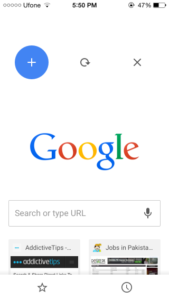Screenshot from a cellphone displaying the home screen. At the very top left, there are five light gray circular icons resembling the letter 'O'. Next to these icons, the word "Uphone" is prominently displayed in black, with the spelling "U-P-H-O-N-E". The time shown on the screen is 5:50 PM and the battery level is at 47%.

Just below "Uphone" on the left side, there is a round blue icon with a white 'X' in the center. In the middle at the top is the refresh button icon, followed by a close icon 'X' on the right. Beneath these icons is the Google logo, immediately followed by the Google search bar.

Further down the screen are two vertical boxes. The first box contains a heading or title labeled "Addictive Tips". The second box below it is labeled "Jobs in Pakistan".